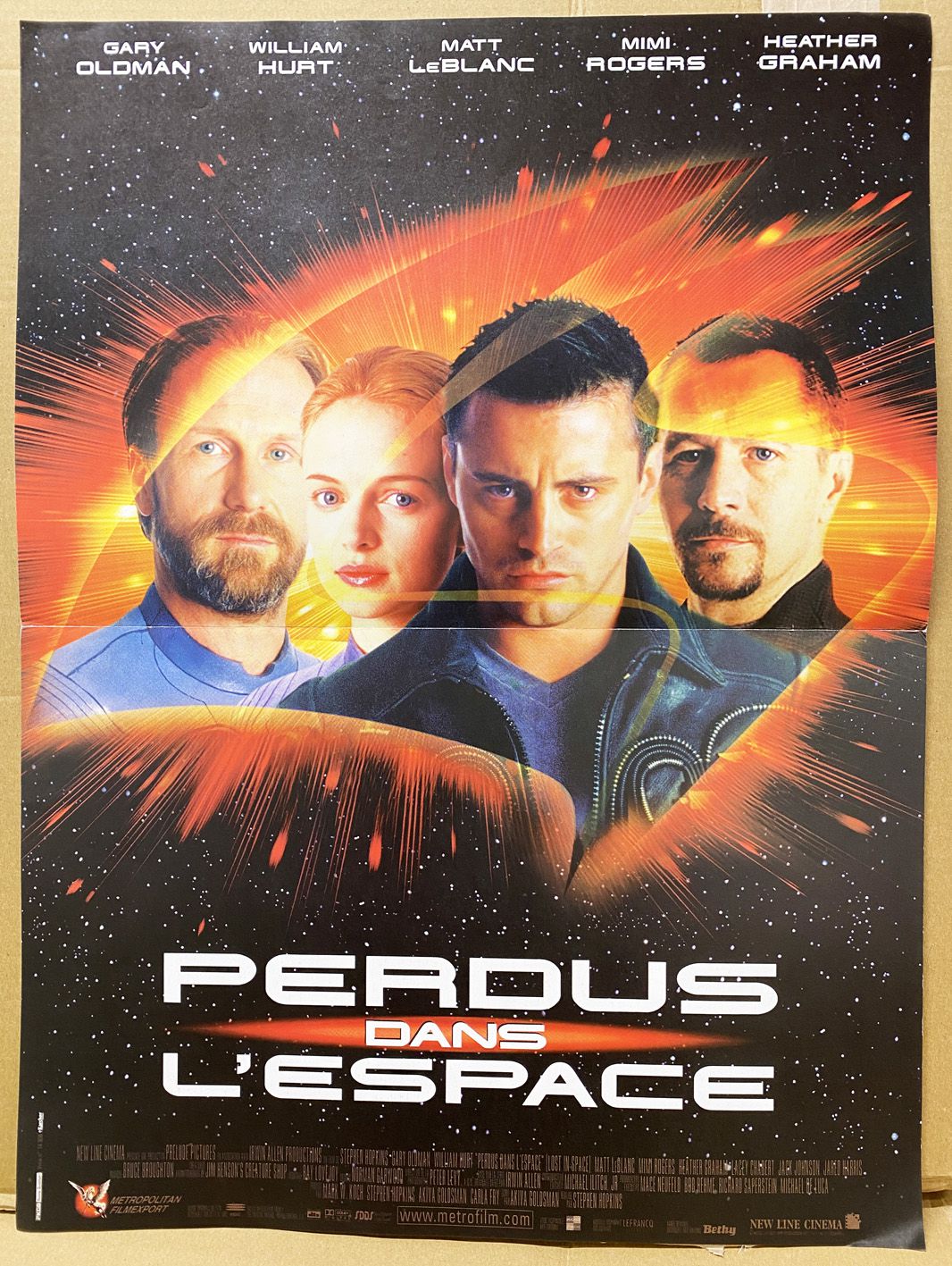The movie poster is an old, visually striking illustration for the film "Perdus dans l'Espace," a French-titled outer space adventure. At the very top, it features the names of the lead actors in bold text: Gary Oldman, William Hurt, Matt LeBlanc, Mimi Rogers, and Heather Graham. Their images are centrally arranged, depicting them against a dramatic space background with a red glow, reminiscent of a sun or other celestial body behind them. The actors are introduced in order from left to right with Gary Oldman, Heather Graham, Matt LeBlanc taking the prominent center position, followed by William Hurt. At the bottom of the poster, the movie's title "Perdus dans l'espace" is prominently displayed in large, white capital letters. Below the title, fine print details the credits, listing the production details. This film is noted to be produced by New Line Cinema, with additional information available at www.metrofilm.com.